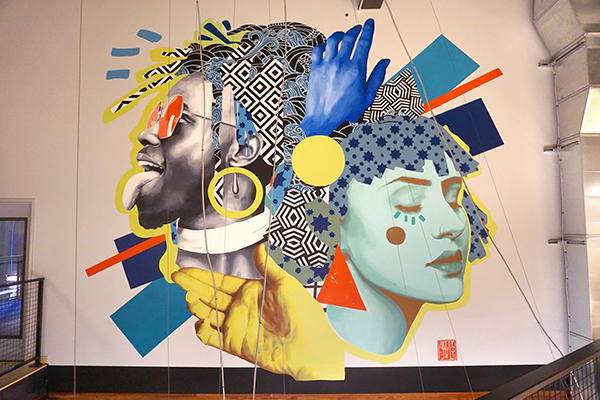The photograph showcases an indoor wall mural, likely situated in a commercial or industrial building and adjacent to a balcony with a mesh-coated railing. The mural spans a towering white wall, potentially reaching at least three stories high. This modern, abstract artwork is vividly colored and features two large, creatively designed heads.

On the left side of the mural is the head of a dark-skinned man. He is depicted in profile with his tongue playfully sticking out, wearing large, red-orange sunglasses, and a bauble earring. Intricate patterns replace his hair, rendered in black and white geometrical designs. A blue rubber glove-like hand extends from the area above his head, creating a striking, detached visual element.

To the right, there is the head of a woman with light green skin, adorned with dark green lipstick, brown eyelashes, and a brown beauty mark on her cheek. Her hair is depicted in blue geometrical patterns, suggesting a sense of flowing contours. A yellow rubber glove hand appears to be holding or supporting the entire composition near the necks of both figures.

Overall, this polychromatic mural combines bright blue, yellow, and green hues, injecting a lively and avant-garde appeal into the space it occupies. The juxtaposition of the two faces with abstract and symbolic elements, such as the rubber gloves and geometric hair designs, contributes to its modern and artistic essence.